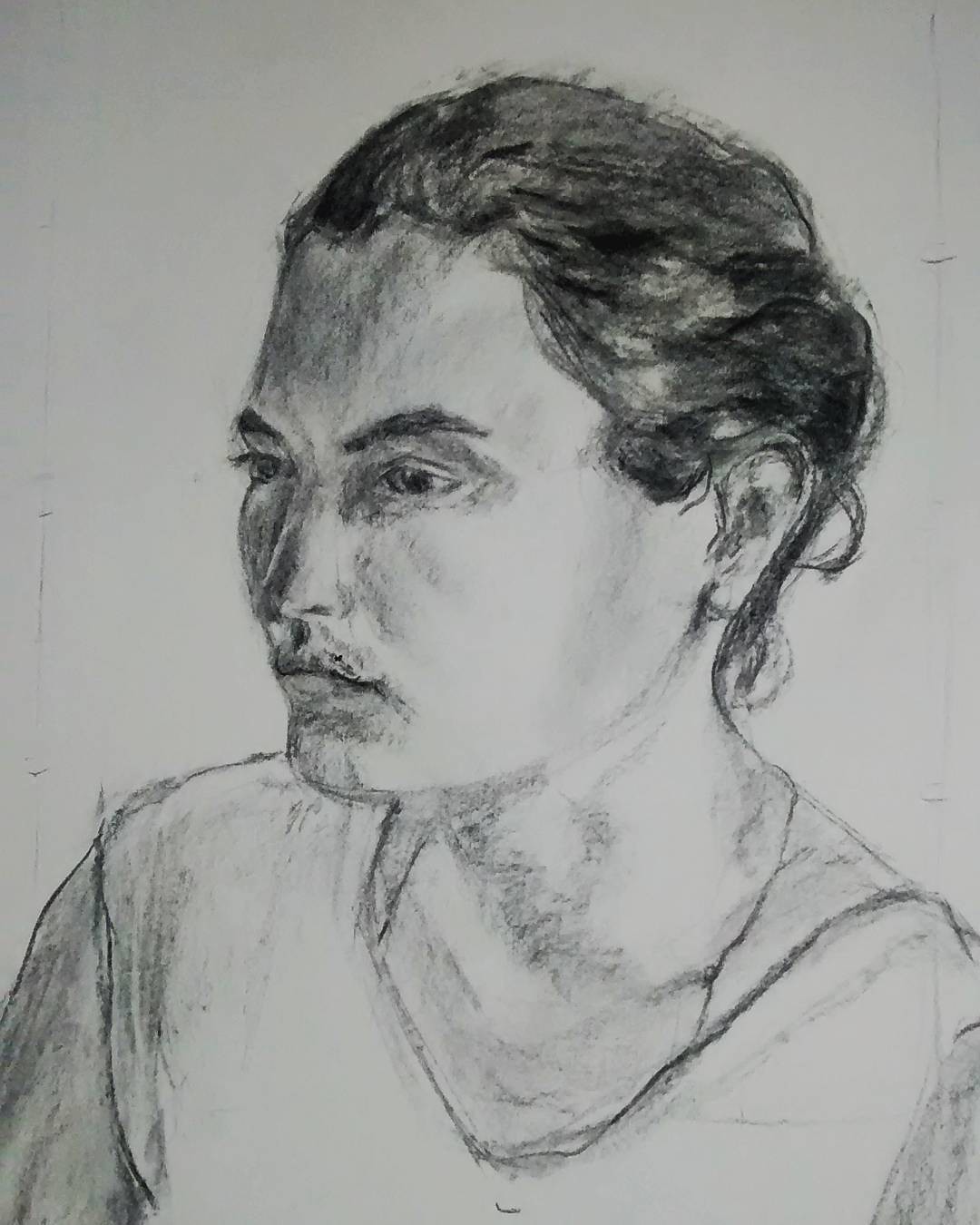An intricately detailed charcoal illustration depicts a pensive figure gazing off to the left, seemingly lost in thought. The artwork features a man with a subtle mustache and goatee, his black hair contrasting against the dauntlessly white canvas. Dressed in a white shirt, the right sleeve appears slightly darker, adding a touch of depth and realism to the piece. The background is enriched with stray, upward marks, enhancing the contemplative mood of the portrait. The central focus remains on the man’s face down to his chest, capturing a moment of introspection suspended in shades of gray and black.